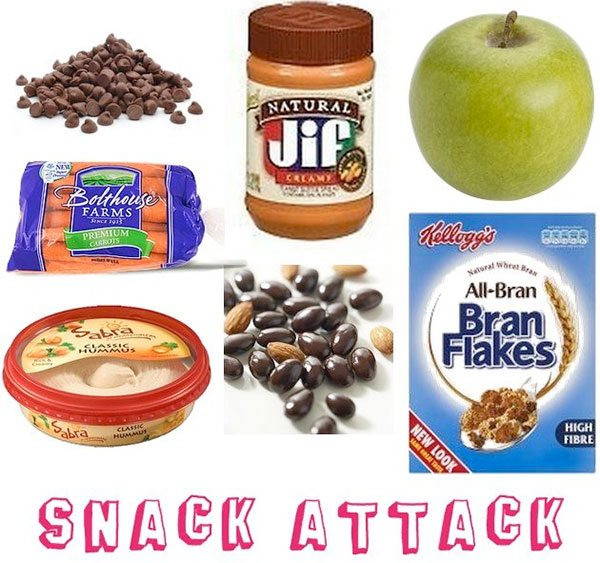The image, entitled "Snack Attack," is a detailed collage of seven distinct food items arranged against a white background with vibrant, 3D text reading "Snack Attack" in white with a pink drop shadow at the bottom. In the upper left corner, there's a loose pyramid of chocolate chips. Moving to the right, there's a brown-lidded jar of Natural Jif creamy peanut butter followed by a bright green apple in the top right corner. Centered in the middle, a bag of Bolthouse Farms carrots is prominently displayed. In the lower left corner, a container of Sabra classic hummus is placed next to a cluster of chocolate-covered almonds and seeds. Lastly, the lower right corner features a box of Kellogg's All-Bran Bran Flakes, complete with a ribbon saying "new look, same great taste." The carefully positioned items, each appearing to be of similar size, create a harmonious and visually appealing layout that emphasizes healthy snack choices.